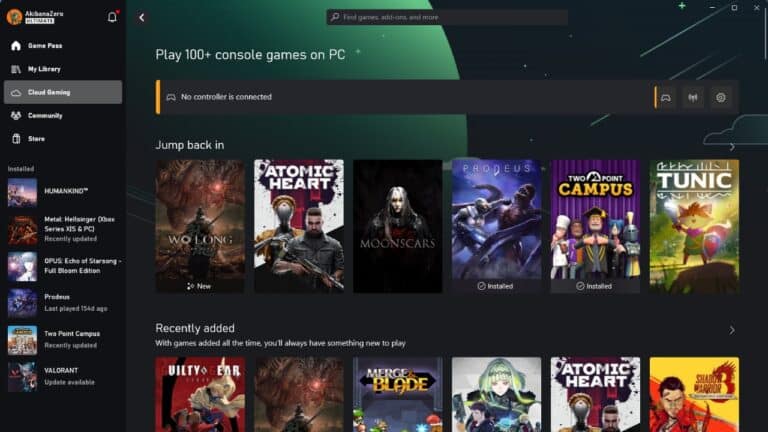Displayed on the right section of the website is a mesmerizing galaxy-themed background, featuring dynamic greenish lines that resemble shooting stars, and a partially visible, misty green cloud. Scattered white dots mimic distant stars, while a prominent, round green mass could be interpreted as a planet. At the top of the page, a functional search bar is positioned, complete with a magnifying glass icon and the prompt: "Find games, add-ons, and more."

In the upper right-hand corner of the interface, control icons are neatly arranged: a dash representing the minimize function, a square for adding a new tab, and a small 'x' for closing the window. Starting from the location of the green planet, bold white text reads: "Play 100+ console games on PC." Beneath this, a dark gray box with a distinctive left orange stripe highlights the notification: "No controller is connected."

Further down, white text prompts the user to "Jump back in," listing various game titles. The featured games mentioned include "Wo Long," "Atomic Heart," "Moonscars," "Prophetess," and a title that appears as "P H-O-D-E-U-S." Additionally, “Utility Gear” is mentioned, though partially obscured, alongside “Merged and Blade” with anime-style imagery. Despite visual clarity issues, "Atomic Heart" is listed once more, and the topmost entry, albeit blurred, seems to be "Shadow Warrior 3."